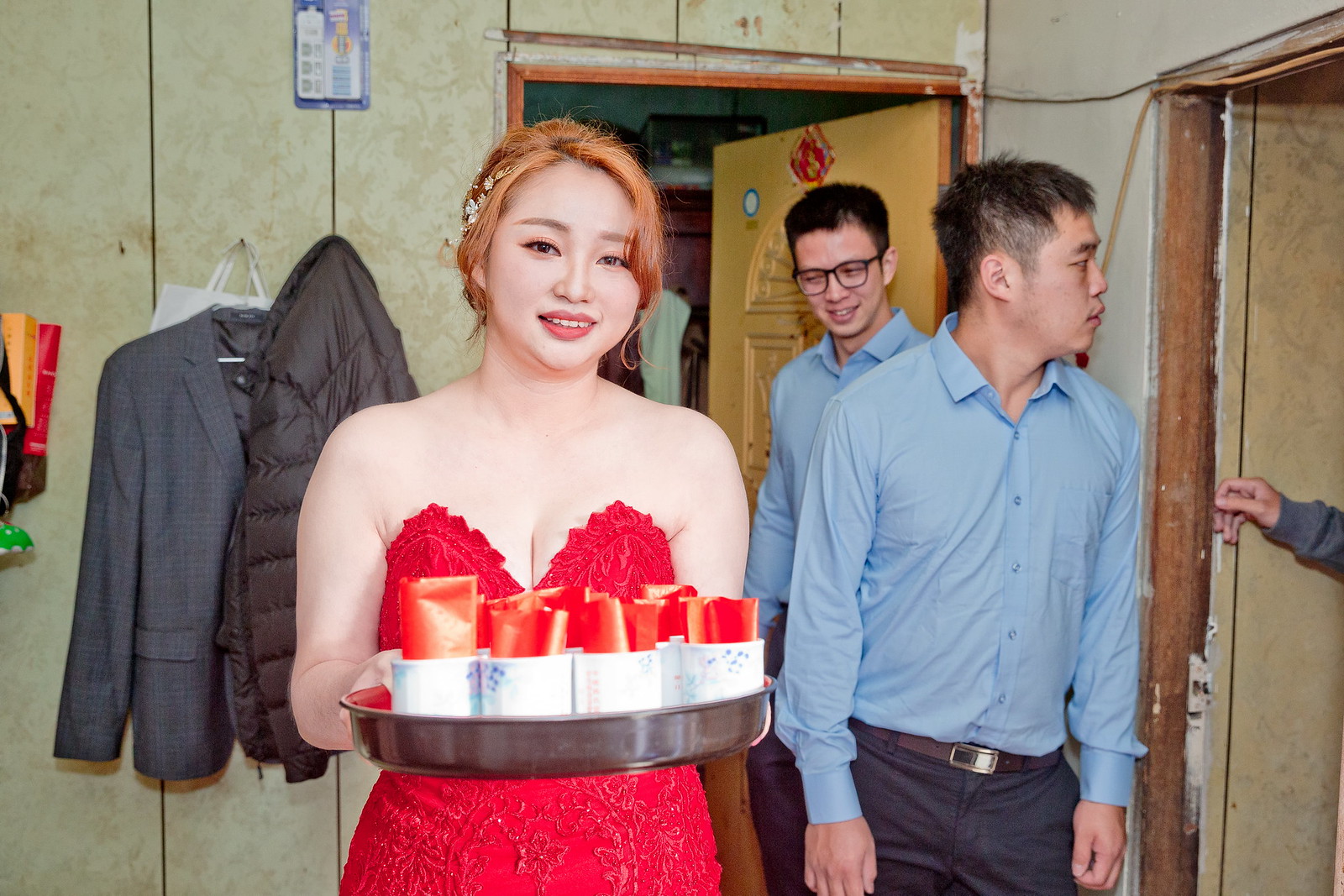The photograph captures a lively scene that appears to be a party or celebration. At the forefront, a young Asian woman, smiling and facing the camera, stands out with her dyed red, ginger-colored hair, most of which is pulled back with flowers adorning it. She wears a strapless red dress and holds a black tray filled with red cartons, possibly containing drinks. Behind her, two young Asian men, seemingly in their early 20s, stand together. Both have closely cropped black hair and are dressed in light blue, long-sleeved, button-down collared shirts. The man closest to the woman wears brown trousers with a brown leather belt and a gold buckle, while the other, slightly behind, wears dark blue trousers and sports dark-rimmed glasses. To the left of the woman, the tan-paneled wall features hooks with a dark gray suit jacket and a black puffy ski jacket hanging from them. Additional details include an interior room setting with two doors; one door behind the men has a glimpse of an arm grasping the frame, and another door in the background adds depth to the celebratory ambiance. The walls feature a subtle floral pattern, further enriching the scene's intricacy.